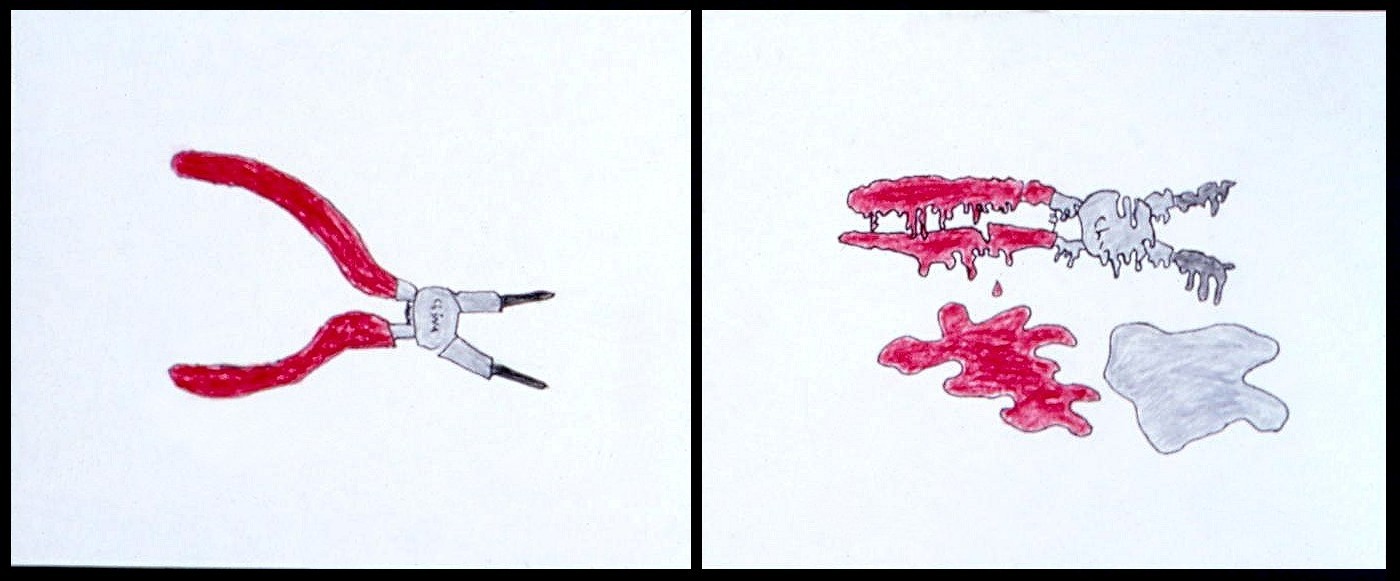The image depicts a pair of side-by-side hand-drawn illustrations on a white background, each enclosed in a narrow black frame. The left drawing features a pair of pliers with red handles, spread apart, and drawn in what appears to be colored pencil or marker. The metallic body and hinges of the pliers are colored in gray, while the grasping jaws, positioned to the right, are shaded in black. The right drawing portrays these same pliers, now appearing as if they are melting. The red handles, closer together, seem to be dripping, with red puddles forming below. The metallic gray part of the pliers is also depicted as melting, resulting in a silver puddle beneath it. This illustration includes disturbing details where the melting pliers suggest blood and a separated tooth, adding a graphic and eerie dimension to the overall depiction. The artwork is vividly colored and clearly rendered, with sharp details highlighting the unsettling transformation of the pliers.